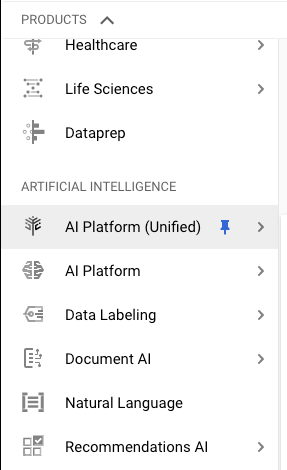The image is a black and white schematic with a white background, featuring various categories and subcategories marked in black or gray text. 

At the top, the first category, "Products," is accompanied by an upward arrow. Below it are three subcategories: 

1. **Healthcare** (with an adjacent black-and-white image and an arrow pointing to the right).
2. **Life Sciences** (with another black-and-white image and an arrow pointing to the right).
3. **Data Prep** (with a black-and-white image but no right-pointing arrow).

Beneath "Products," there is a section labeled "Artificial Intelligence." Within this section, there is a gray-highlighted box labeled "AI Platform (Unified)" with a blue thumbtack icon beside it and an arrow pointing to the right. 

Further down, additional categories listed are:

- **AI Platform** (with an arrow to the right)
- **Data Labeling** (with an arrow to the right)
- **Document AI** (with an arrow to the right)
- **Natural Language** (no arrow)
- **Recommendations AI** (with an arrow to the right)

Each of these categories on the left-hand side is accompanied by images or symbols.

The layout suggests the possibility of scrolling up or down to view more content, as implied by the structured listing.